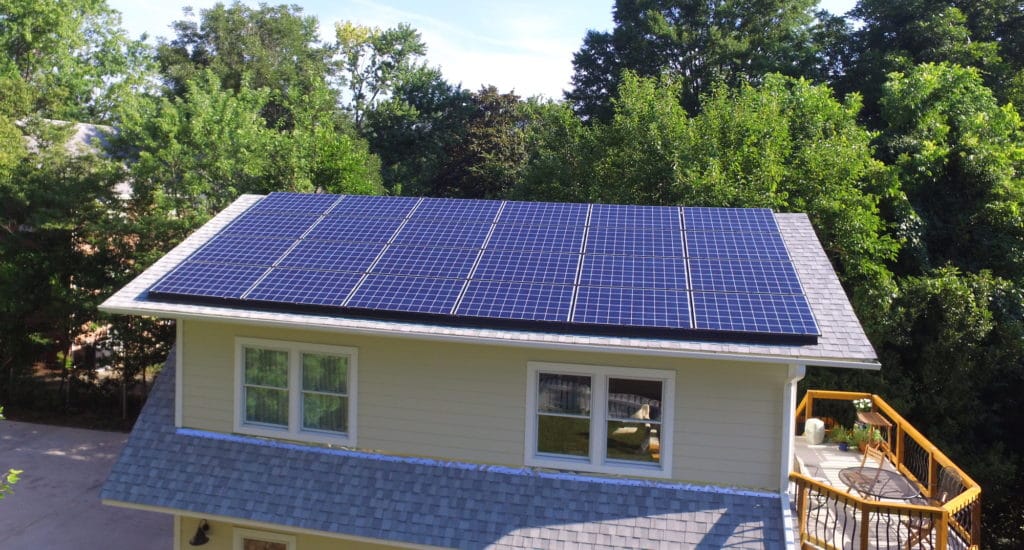The image showcases a two-story house with a flat, gray roof adorned with an array of solar panels. The panels are arranged in a meticulous grid comprising six columns and four rows, each panel displaying a series of smaller square cells in a vibrant blue hue. The house itself is painted a subtle whitish-yellow, contributing to its charming aesthetic. 

On the right side of the house, there is a deck featuring a brown wooden railing, furnished with several small chairs and a metal table, suggesting a quaint outdoor seating area. To the left, a driveway with a white-gray surface is visible. Surrounding the house is a lush landscape filled with various green trees and dense foliage, enhancing the serene and picturesque atmosphere of the setting. The sky above is a clear blue with patches of white clouds, indicating a bright and sunny day.